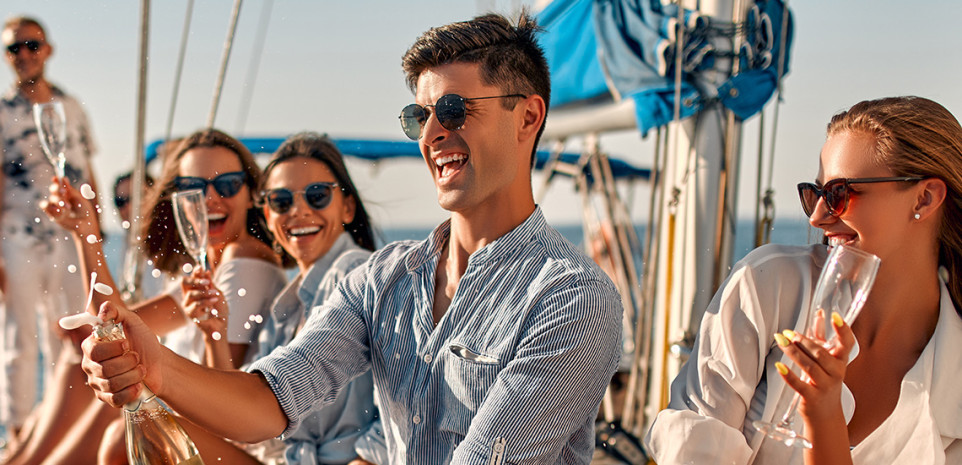A vibrant, horizontal color photograph captures a lively yacht party with a group of animated individuals who appear digitally rendered, suggesting the use of Photoshop. In the foreground, a tan, excited man takes center stage, dressed in a blue and white pinstripe shirt and sporting sunglasses. With his mouth open in exhilaration, he is dramatically popping open a bottle of champagne. Behind him, two women, also wearing sunglasses, hold up their champagne glasses, smiling and laughing, exuding a sense of joy and festivity. On the left edge, a smiling man contributes to the energetic atmosphere, while on the right, a woman with striking bright yellow nails gazes intently at the champagne bottle, her glass poised in her hand. The scene is bathed in sunlight, casting pronounced highlights and shadows that enhance its surreal, artificial appearance. This image masterfully conveys the essence of a high-spirited celebration, albeit through a lens that blurs the line between reality and digital artistry.